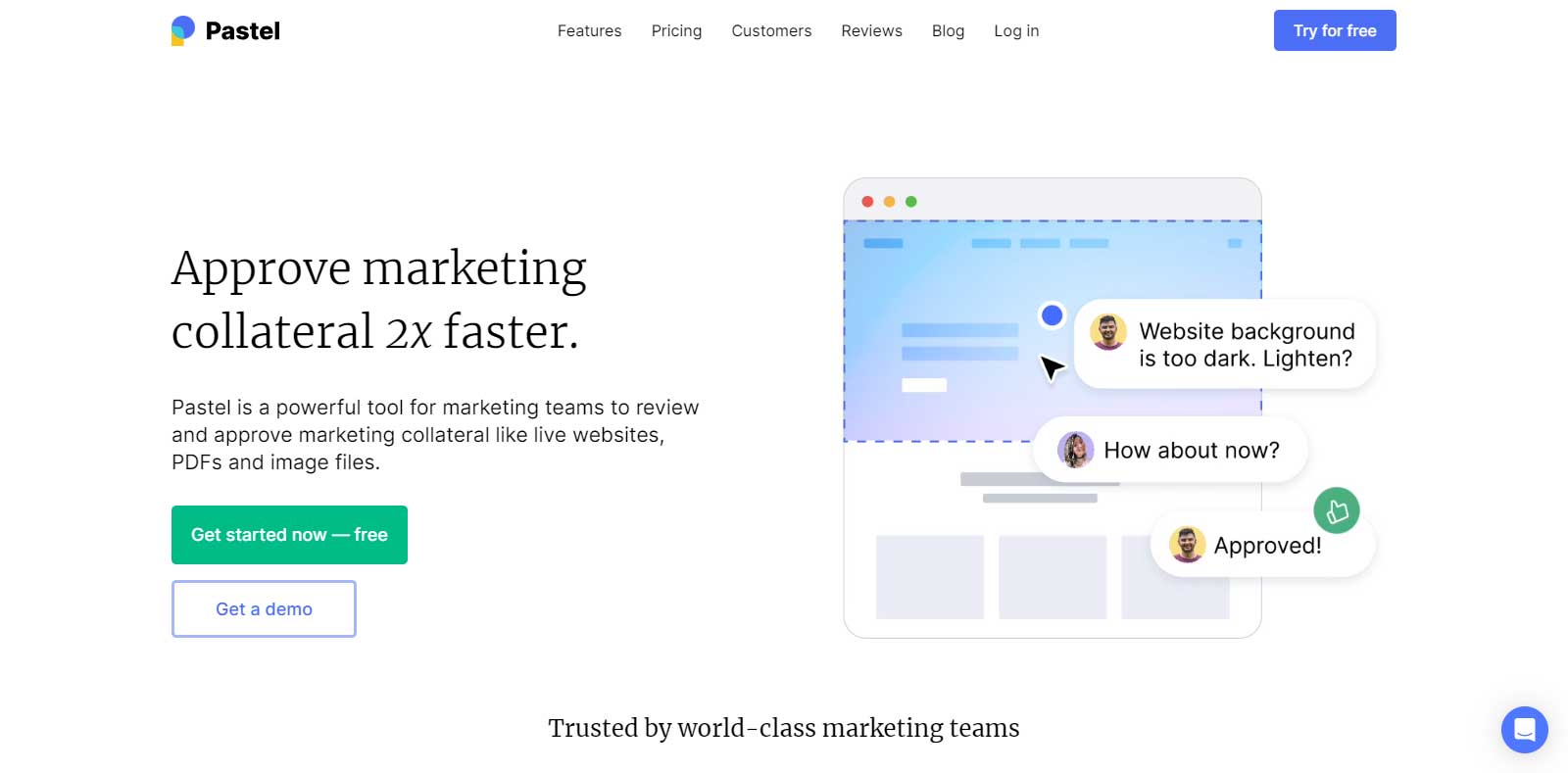The image is a horizontally rectangular screenshot from a website with a white background. In the top left corner, the website name "Pastel" is displayed, accompanied by a small logo to its left. Centered on the top navigation bar, there are several options: "Features," "Pricing," "Customers," "Reviews," "Blog," and "Login." On the far right, a prominent blue button with white lettering reads "Try for Free."

The main content of the page is divided into two sections. On the left, there is a headline that states, "Approve marketing collateral 2x faster." Below this headline, a brief description explains that "Pastel is a powerful tool for marketing teams to review and approve marketing collateral like live websites, PDFs, and image files." Beneath this description, two buttons are displayed: a green button labeled "Get Started Now Free" and a white button outlined in blue labeled "Get a Demo."

On the right side of the image, there is a rough outline of a webpage with no specific details. Overlaid on this outline are speech bubbles with avatars. The text within these bubbles includes, "The website background is too dark, lighten," with a response saying, "How about now?" and then another response stating, "Approved."

At the bottom center of the image, a statement reads, "Trusted by world-class marketing teams."